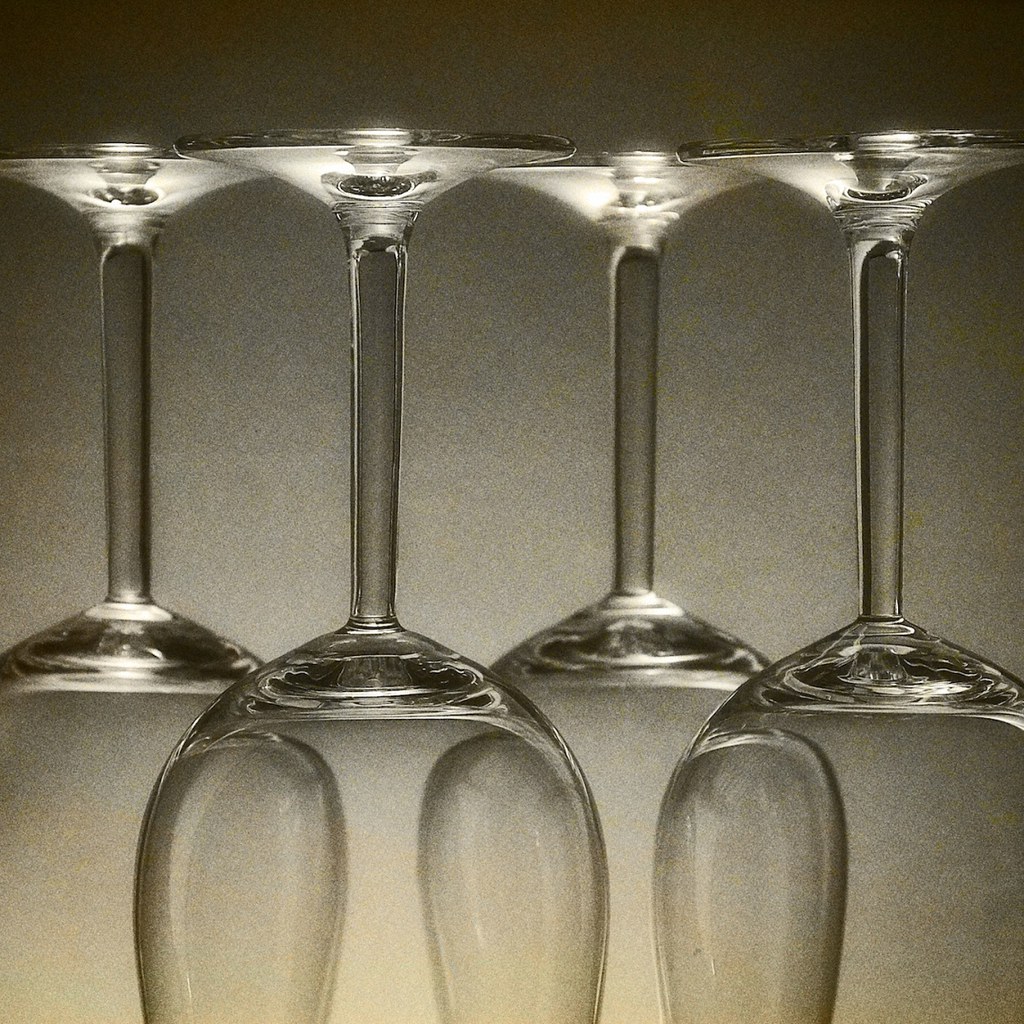The image is a close-up, black and white photograph of four upside-down wine glasses, arranged in a visually striking, overlapping pattern. The glasses, possibly made of glass or crystal, are positioned in two rows: two in the front and two in the back, slightly offset from each other. The stems of the glasses are notably long, and their bases exhibit bright, white highlights due to reflections. The background features a gradient that transitions from a deep gray at the top to a lighter shade, and faintly exhibits a yellowish hue at the bottom. The image has a grainy texture, adding to its artistic quality. The scene is highly evocative, with the translucent and polished surfaces of the glasses creating a dynamic interplay of light and shadow.